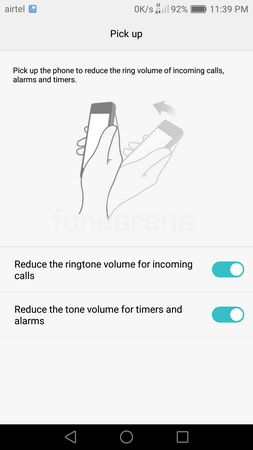This image appears to be a cell phone screenshot, with dimensions approximately 2.5 times taller than it is wide. It showcases an app interface. 

At the top of the screenshot, the status bar displays "Airtel" on the upper left and "0 K/s" on the upper right, alongside a low signal strength icon. The battery indicator shows 92% with an almost full battery icon, and the current time is 11:39 p.m.

The background is a light gray, and centered near the top of the screen is the text "Pickup" in black. Below that, in smaller black text, it reads "Pick up the phone to reduce the ring volume of incoming calls, alarms, and timers." 

The visual beneath the text depicts an instructional graphic with a hand holding a phone at the 12 o'clock position, and a second, semi-transparent outline of the hand holding the phone at approximately the 1:30 position. An arrow points from the right image (1:30 position) to the left one (12 o'clock position), illustrating the motion of picking up the phone.

Below the graphic, two options are listed: "Reduce the ringtone volume for incoming calls" and "Reduce the tone for incoming timers and alarms." Both options are toggled on.